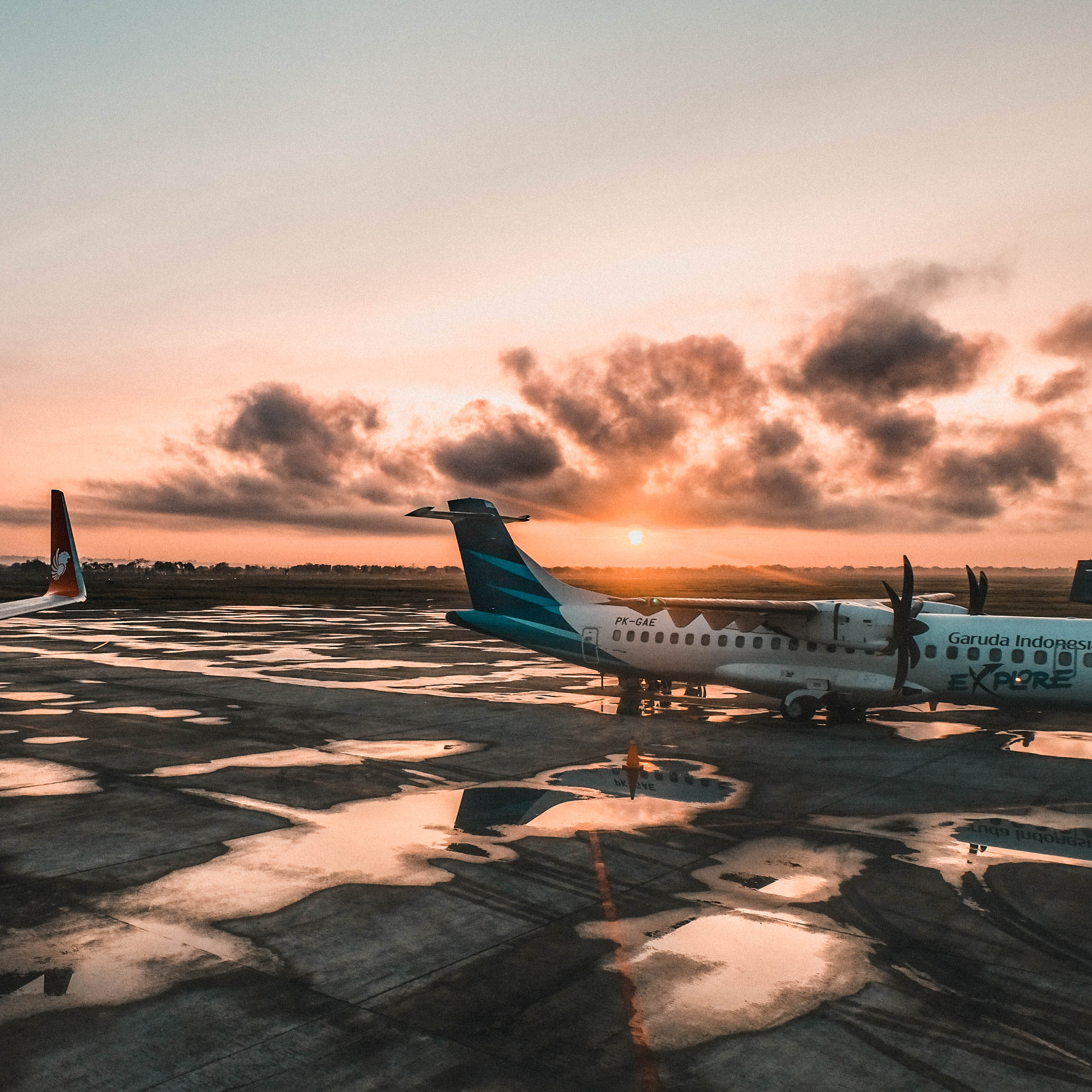The photo captures the scene of an airplane hangar against a post-rain, twilight sky. The ground is cemented with scattered water puddles, reflecting the recent rainfall. In the foreground, there are two airplanes partially visible; the airplane on the right has most of its body shown and features a white exterior with a blue tail marked with the text "Garuda Explore PK-GAE." This plane has propellers that resemble the shape of palm trees. The airplane on the left is only visible by its tail, which is painted red. The dominant colors in the scene include white, black, various shades of blue and brown, and touches of red. The sky above features a mix of gray clouds with a sun peeking through in an orange hue, creating a striking backdrop for the scene below. İn the middle distance, patches of dirt and silhouettes of trees can be seen beneath the setting or rising sun, casting a reddish glow across the sky.